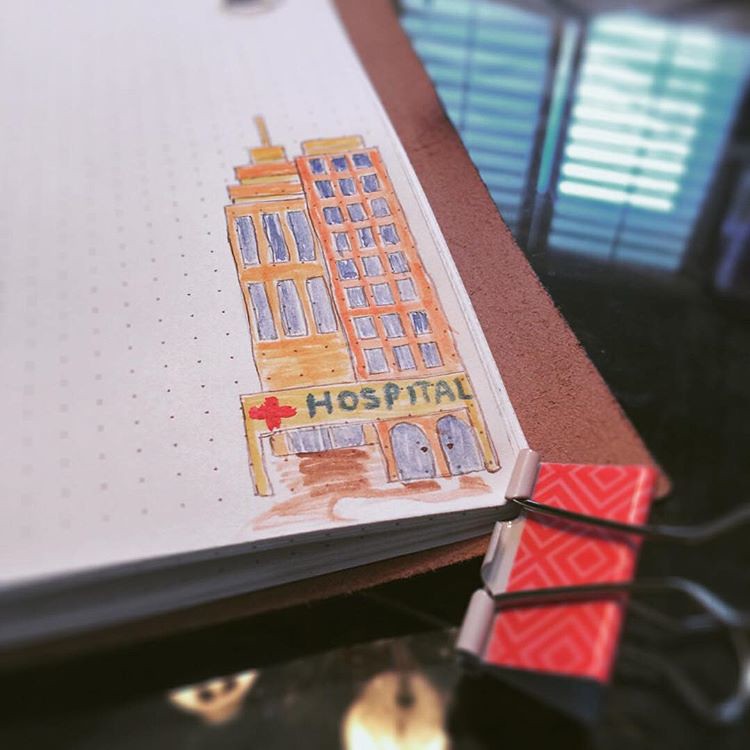The photograph captures a detailed portion of a drawing situated in the bottom right corner of a page within an open notebook, possibly brown leather-bound. The paper has a dotted grid pattern running vertically across the entire page. The drawing appears to be of a hospital, likely created by a child using crayons or markers. The hospital is depicted as two tall, brown buildings, one slightly lighter than the other, adorned with numerous blue-colored windows. At the top of the left building, there is a spiral feature capped by a tower. The word "hospital" is prominently displayed along the bottom edge of the drawing, accompanied by a red cross typically associated with medical facilities. There are two purple-doored entrances shown on the drawing. The page is clipped to a black clipboard and remains attached to the notebook, with several visible pages beneath it. The notebook rests on a glass table, reflecting the overhead light and windows with open blinds to the right.